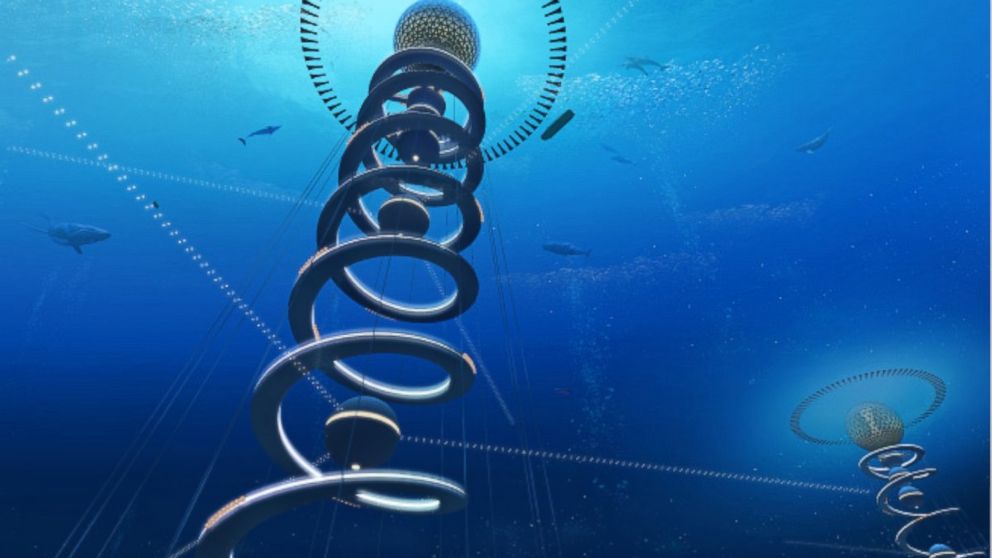The image depicts a detailed, simulated underwater scene, dominated by an advanced high-technology structure. The environment is imbued with blue tones, reminiscent of deep ocean or aquarium settings. Toward the center of the image is a towering metal coil that spirals upward from the dark depths to the brighter surface. This coil encompasses several sections with blue balls adorned with a cream-colored stripe. Topping the coil is a distinctive polyhedral yellow ball, encircled by black dashes forming a partial concentric ring, partially cut off by the image's upper boundary. There is also a smaller similar coil in the bottom right corner, further down and fully visible with its complete circular markings. The scene is populated by large sea creatures, including fish and possibly whales, swimming amidst the structure. Light sources seem to emanate from above, illuminating the structure and creating a striking interplay between light and shadow as it pierces through the water. The entire setup gives an impression of an otherworldly or alien underwater high-tech installation.